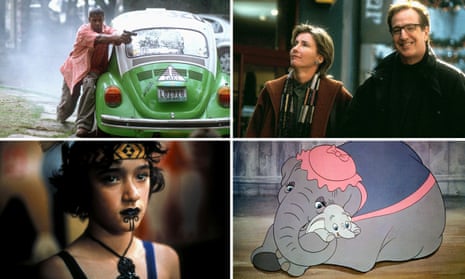The image is a collage of four movie stills arranged in two rows and two columns. The top left photograph features a dramatic scene in a misty forest where a man, possibly African American, leans against an old, green Volkswagen Beetle with a white top. He is dressed in a white and red cardigan and holds a gun in each hand, appearing alert and ready to shoot. The top right image depicts a cheerful moment in front of a store, showing a man with glasses, smiling widely, dressed entirely in black. Beside him is a blonde woman with an upward gaze, adorned in a brown jacket, and likely wearing a scarf. This image suggests a Christmas-themed movie. The bottom left photograph presents a young androgynous individual with black curly hair, dark lipstick, a chin tattoo, and a dark blue tank top, suggesting a rebellious or alternative vibe. Finally, the bottom right image is an animated still from "Dumbo," showcasing a tender embrace between Dumbo and his mother, with his mother donning a pink hat.